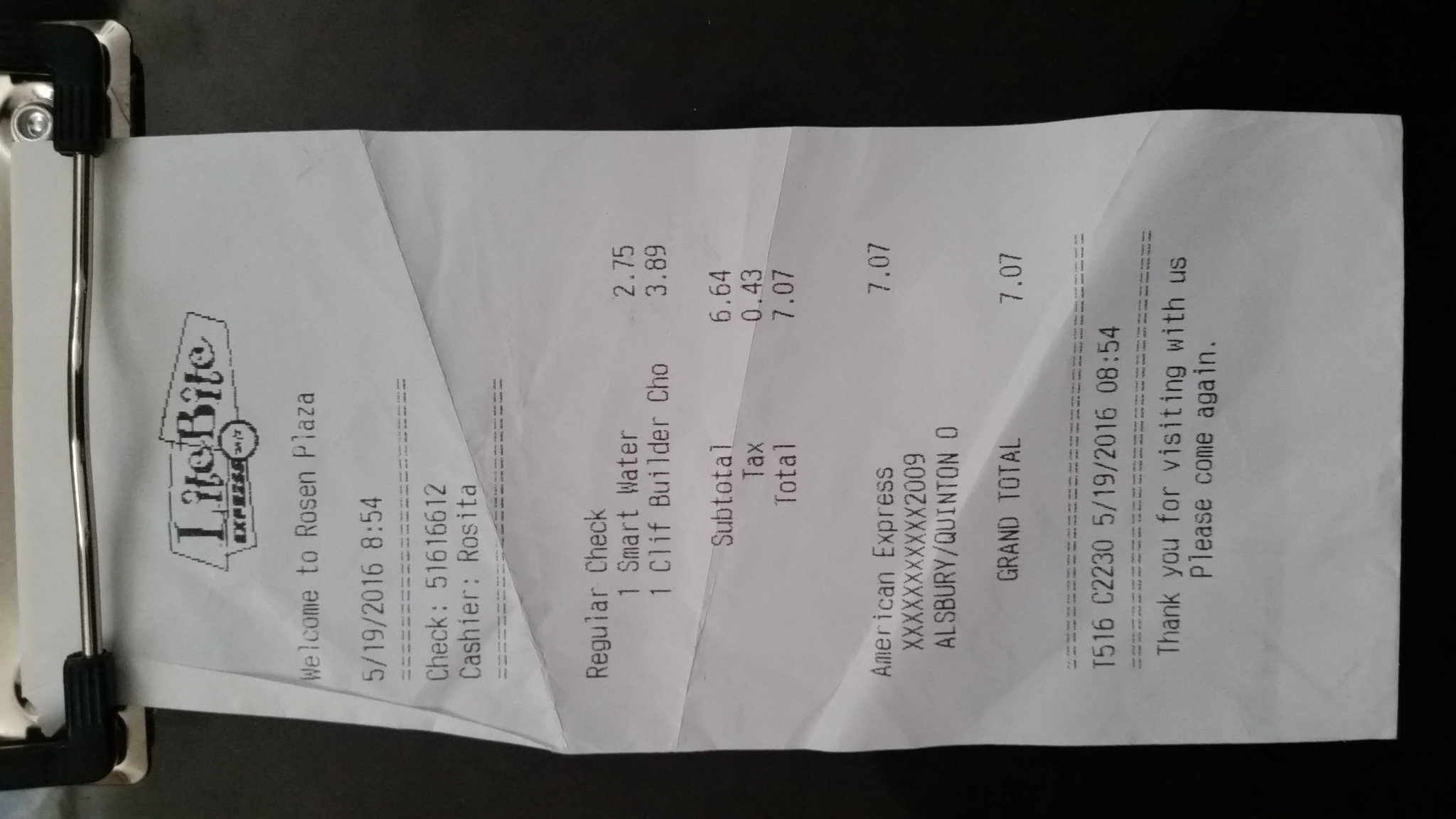This image captures a slightly wrinkled receipt clipped to a black clipboard with a metal clip, positioned sideways on a white paper background. The receipt is from "Light Bite Express," a 24/7 store located in Rosen Plaza, dated May 19, 2016, at 18:54. The cashier's name is Rosita. The purchased items listed are one Smart Water and one Clif Builder chocolate bar, totaling $7.07, paid with an American Express card. The receipt also includes a courteous message saying, "Thank you for visiting with us. Please come again."